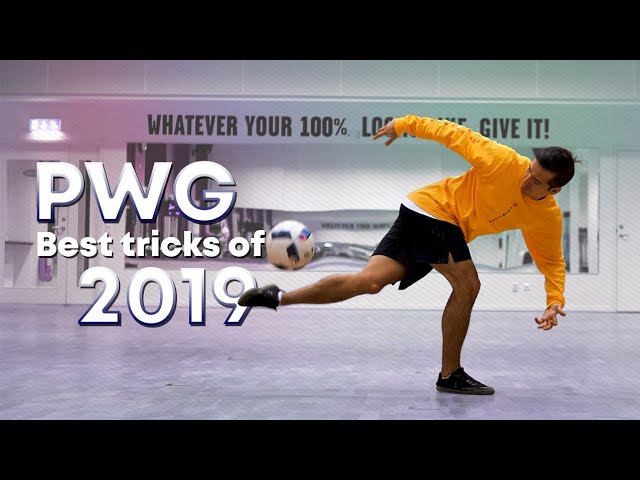This image captures a dynamic moment featuring a man performing a soccer trick, set within what appears to be a spacious gym or workout room. The man is dressed in a long-sleeve orange shirt, black shorts, black sneakers, and white socks. His black hair frames his focused expression as he kicks a soccer ball with his left leg extended behind him. In the background, a partially obscured motivational quote on the wall reads, "Whatever your 100% ... give it!" The overall scene is framed with black bars at the top and bottom, typical of a screenshot from a video. Prominently displayed in big white letters are the words "PWG best tricks of 2019," indicating this image is from a video showcasing impressive soccer skills.